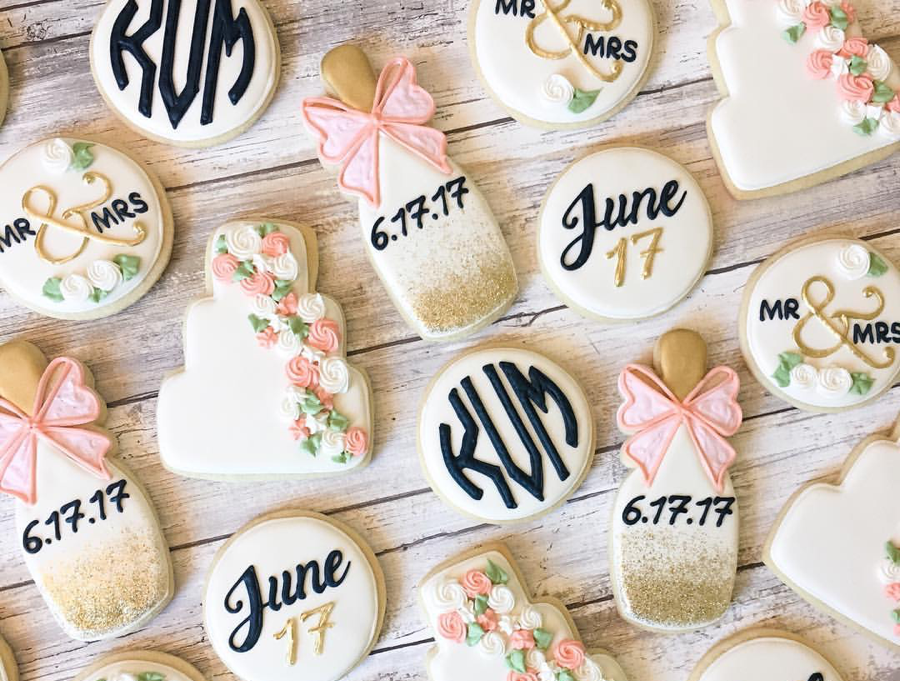The photograph, taken indoors, is rectangular in shape and measures approximately six inches wide by four inches high. The background features a shabby chic style with whitewashed wooden slats arranged diagonally from the lower left to the upper right. The image predominantly showcases an assortment of intricately decorated cookies, suggesting a marriage theme. 

The cookies come in various shapes: circles, wine bottles, and a three-tiered wedding cake. The wine bottle-shaped cookies are adorned with gold icing at the top and bottom, white icing in the middle, and pink bows. They also bear the date "6.17.17" in black icing. The circular cookies are iced in white and feature different inscriptions, such as "June 17" in gold, "KVM" in black, and "Mr. and Mrs." in black. 

The three-tiered cake-shaped cookies are detailed with white and pink roses, complete with green leaves. All the cookies are arranged artistically across the whitewashed wooden background, creating a cohesive and visually appealing display centered around a marital celebration theme.